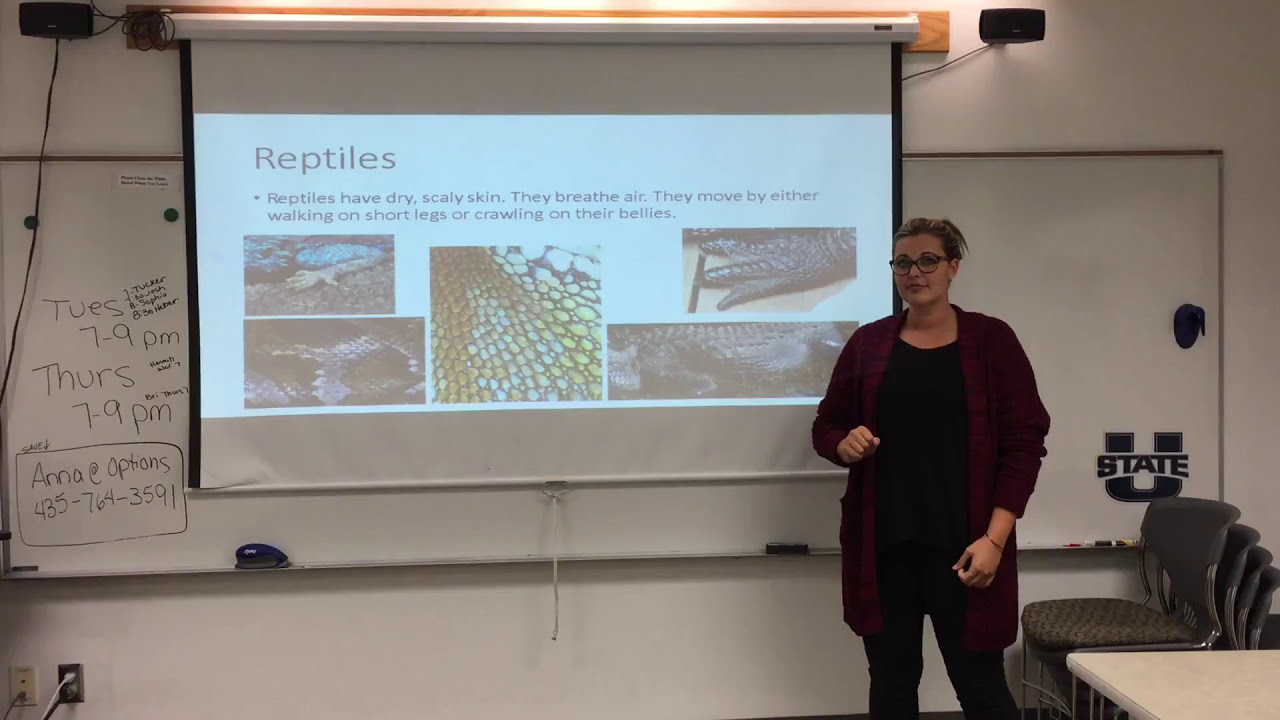The image captures the inside of a classroom with solid white walls, dominated by a large white dry erase board mounted on the back wall. To the left side of the board, there is a schedule written in black marker that reads "Tuesdays 7 to 9 p.m." and "Thursdays 7 to 9 p.m." Beneath the schedule, it says "Anna at options" followed by the phone number 535-764-3591. On the lip of the dry erase board, there is a marker and two erasers. The right side of the board features a sticker that says "State U."

In front of this scene is an overhead projector screen displaying a slide about reptiles, which highlights that reptiles have dry, scaly skin, breathe air, and move either by walking on short legs or crawling on their bellies. Various images of reptiles are depicted below the text. Standing in front of the screen is a lady facing the viewer, dressed in a black outfit with a red sweater, wearing glasses, and her hair tied up in a bun. 

The meticulous attention to details such as the room's white walls, the content on the dry erase board, and the educational slide on reptiles, creates a vivid depiction of a classroom setting, emphasizing the learning environment and schedule.